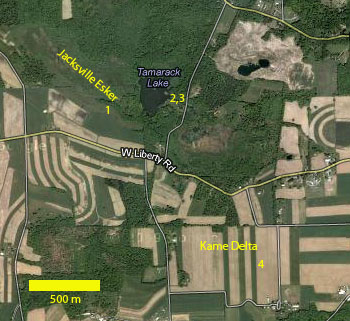The image is of a satellite view map displaying a top-down perspective of a varied landscape featuring land and water elements. In the top left corner, there's a labeled area called "Jacksville-Esker" with a number "1" beneath it. To the right of this area, a small lake named "Tamarack Lake" is shown, featuring the numbers "2, 3" below its label. In the bottom right corner, "Kame Delta" is marked with a number "4" next to it. The map features a significant amount of greenery interspersed with brown patches, possibly agricultural land or uncultivated areas. There are also various roads visible, with some labeled in white and others in bright yellow, including "West Liberty Road." The bottom left corner of the map includes a yellow horizontal bar, indicating a scale of "500 M." The map's appearance suggests it might have been pieced together, as it looks somewhat fragmented and artificial, highlighting topographic features and both man-made and natural elements.